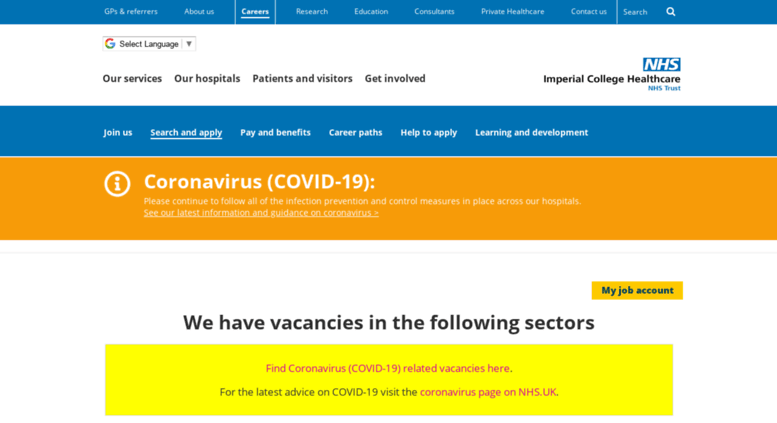The image displays the Careers page of the Imperial College Healthcare website. At the top, a navigation bar features various clickable tabs labeled as follows: "About Us," "Careers," "Research," "Education," "Consultants," "Private Healthcare," "Contact Us," and a search icon symbolized by a magnifying glass. To the right of these tabs, there is a drop-down menu with a Google icon that allows users to select their preferred language.

Below the primary navigation bar, secondary tabs provide further options, including "Our Services," "Our Hospitals," "Patients and Visitors," and "Get Involved." Below these, a blue banner highlights several additional navigation links: "Join Us," "Search and Apply" (which is the current tab and is underlined for emphasis), "Pay and Benefits," "Career Paths," "How to Apply," and "Learning and Development."

Beneath the blue banner is a prominent dark orange banner featuring an eye icon, which provides important COVID-19 information. The banner reads: "Coronavirus (COVID-19). Please continue to follow all the infection prevention and control measures in place across our hospitals. See our latest information and guidance on Coronavirus."

Following the orange banner, there is additional text indicating the availability of job vacancies across various sectors. It also directs users to find Coronavirus-related updates and advises visiting the Coronavirus page on NHS.UK for the latest COVID-19 advice.